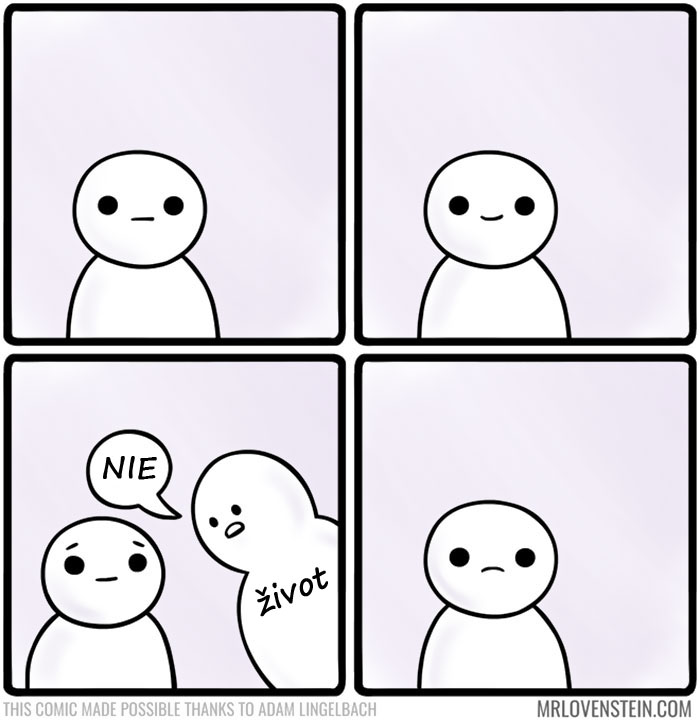The image features a four-panel comic strip with simple line drawings of a stick figure character. The first panel, located at the top left, depicts the main character with a round face, two dot eyes, a straight horizontal line for a mouth, and no arms, presenting an emotionless expression. In the second panel, at the top right, the same character appears with a slight smile, indicated by a small upward arc for a mouth. The third panel, situated at the bottom left, introduces a second character wearing a T-shirt that reads "Zivot" with a diacritical mark on the 'Z'. This new character is looking down at the original figure while saying "NIE" in a speech bubble. The original character now has eyebrows and appears pensive. In the fourth and final panel, located at the bottom right, the second character exits, leaving the original figure frowning. Below the comic, in small gray letters, it reads "This comic made possible thanks to Adam Lingelbach" on the left, and "mrlovenstein.com" on the right. Each cell is bordered by a thick black line.